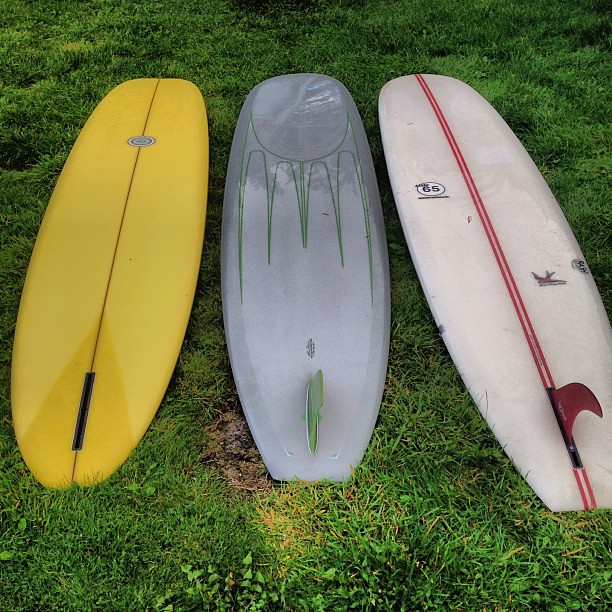The photograph depicts three surfboards lying side by side on a well-manicured, green grassy ground. The entire scene is captured outdoors with no visible sky, focusing entirely on the surfboards and the grass. 

On the left, there is a yellow surfboard with a distinctive red stripe running up the middle. About two-thirds of the way up from the bottom, there is a circular icon featuring a gray design.

The middle surfboard is a dark gray color with lighter gray towards the bottom. It has a green fin facing towards the camera and features a unique design that includes a swirling half-circle pattern with green, dripping lines.

On the right is a white surfboard, marked by two parallel red stripes down the center. It has a red fin and a circular logo that displays the number '65' in black, approximately two-thirds up from the bottom. To the right of the red stripes, there's a small logo resembling a whaling icon.

All three surfboards are well-positioned on the grass, capturing the essence of a beautiful, sunny day.